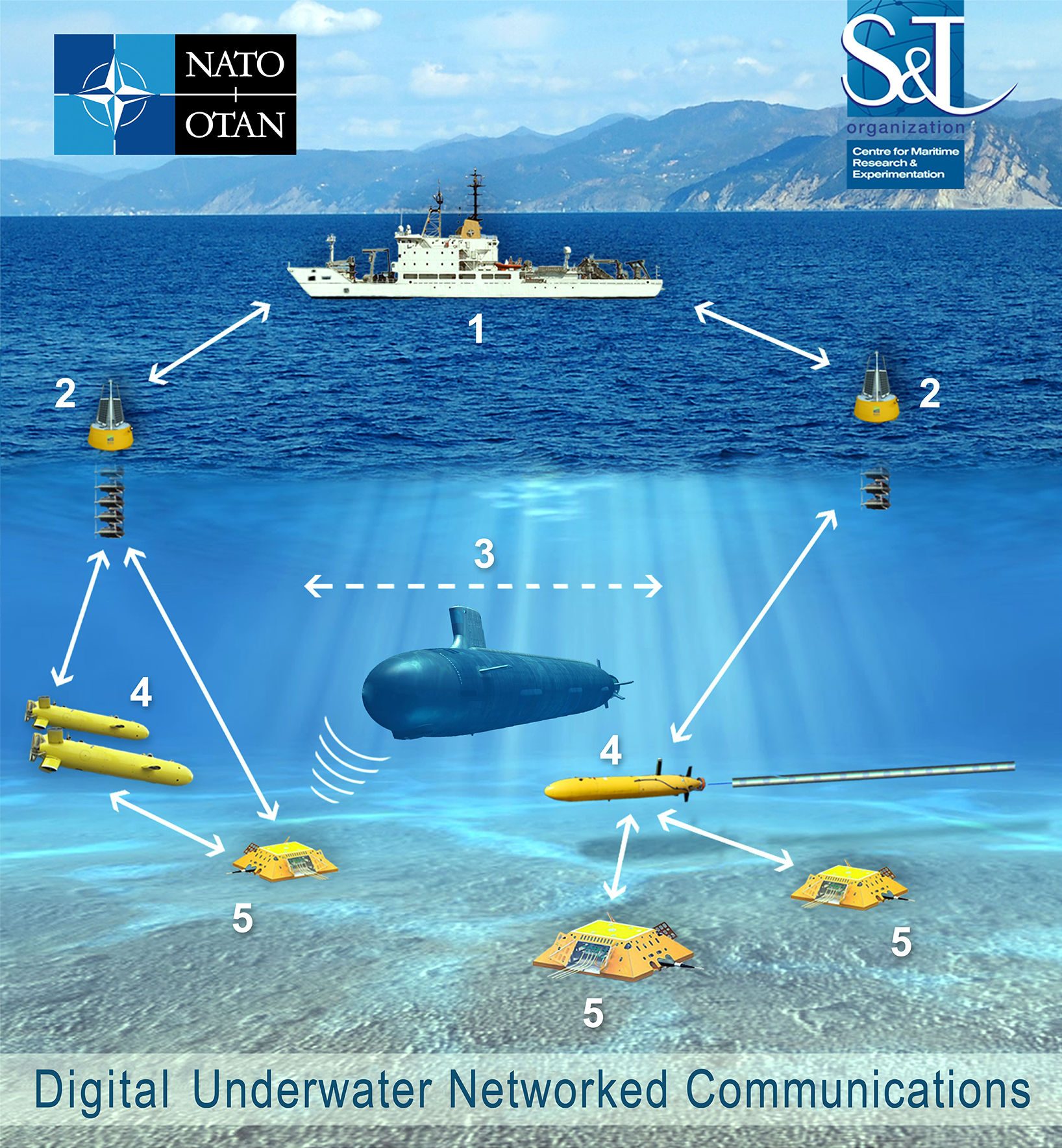A detailed and descriptive caption for the image could be:

"In this intricate poster titled 'Digital Underwater Network Communications,' a vivid underwater scene is depicted with various elements labeled. At the bottom, a gravelly seabed extends, contrasting with the blue waters above. Anchored amid these depths is a large blue submarine. Near the ocean's surface, a pristine white ship navigates the waters. Past the ship, a range of brown and beige mountains rise majestically under a clear blue sky adorned with scattered clouds. The poster features multiple numbered indicators and arrows: '1' points to the ship; '2' directs attention to a floating object in yellow and gray; '3' designates the width of the submarine; '4' points to a smaller, yellow mini-submarine; and '5' identifies a rectangular device, possibly for signal reception, with three instances marked. Additionally, there are two labels numbered '4', emphasizing the smaller submersibles."